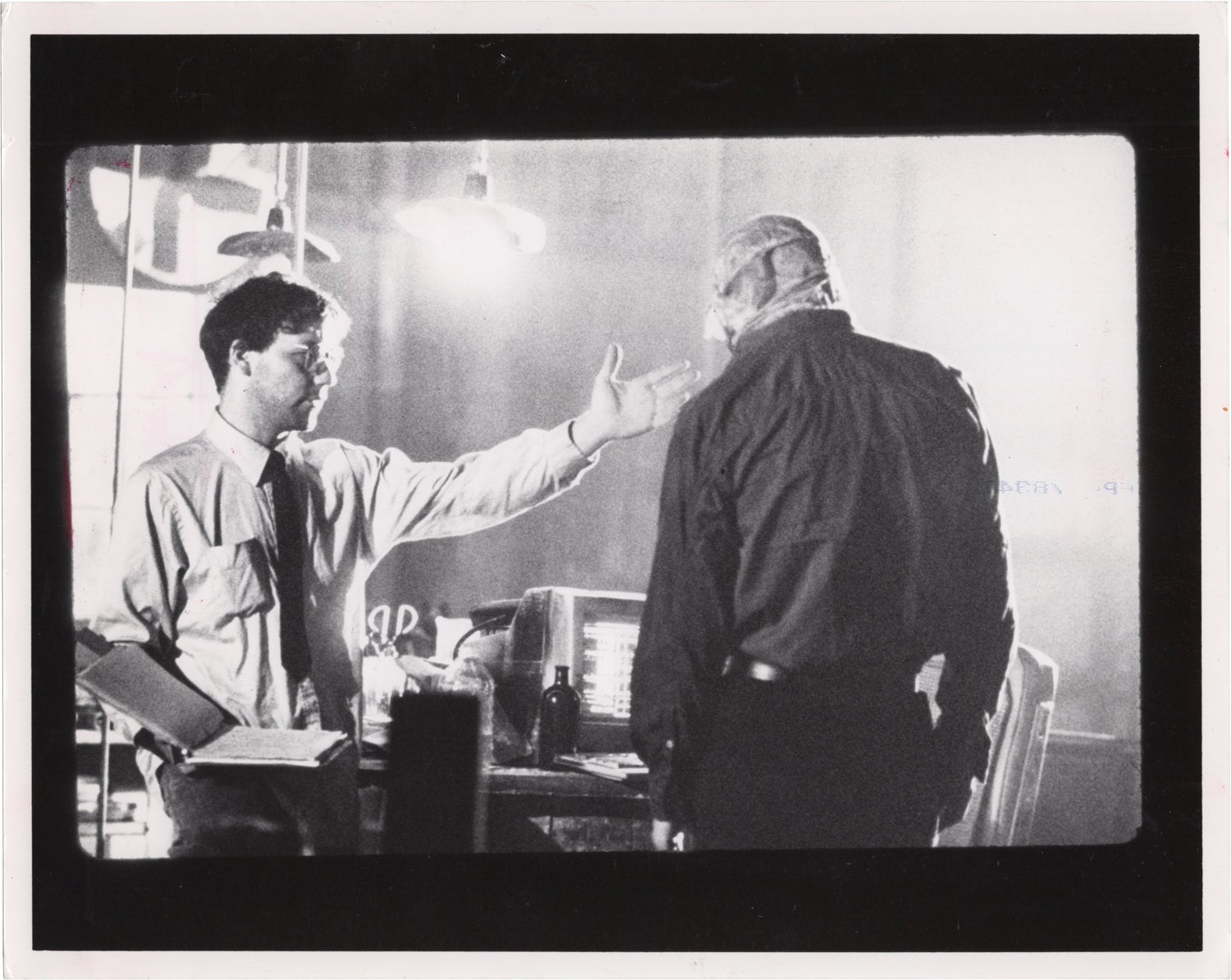The black-and-white image appears to be a still frame from an old science fiction or monster movie. It features a man in a buttoned shirt and a black tie, facing us but with his head turned to the left. He is holding an open binder with papers in his right hand and gesturing toward another man. This second man stands taller and has his back to the camera, dressed in dark pants, a black belt, and a dark, buttoned-up collared shirt. His face, either masked or appearing mutilated, adds to the eerie atmosphere, suggesting he could either be a monstrous creation or heavily disfigured. The setting includes two hanging lamps, reminiscent of inexpensive warehouse lights, adding to the vintage or industrial feel. On a desk in the background, there's an old-fashioned computer monitor, a dark bottle, and scissor-like objects, further hinting at a laboratory environment. The scene suggests an interaction between a scientist and his creation, blending elements of horror and science fiction.